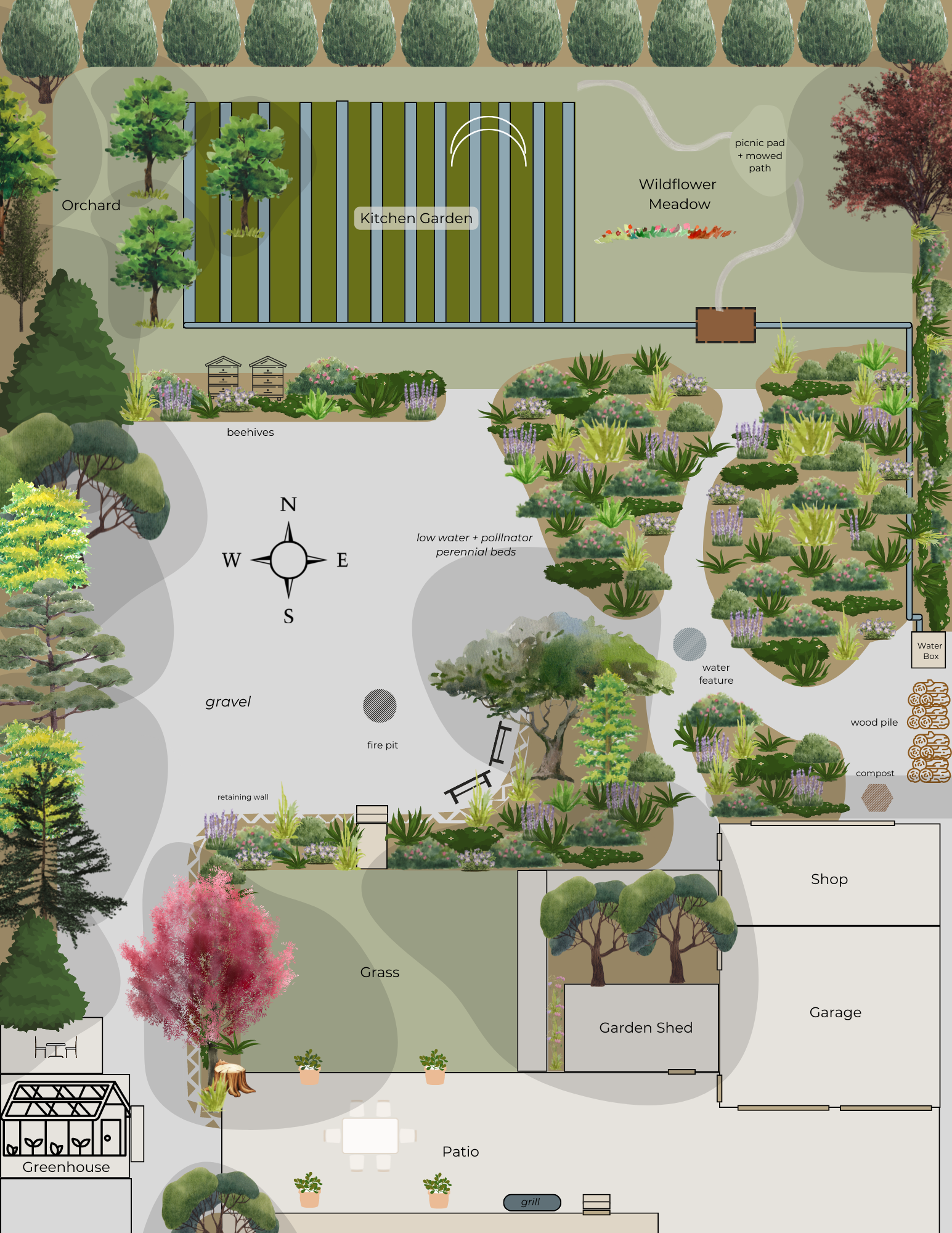The image portrays a detailed, hand-drawn map in portrait mode, illustrating a lush, expansive garden layout. At the very top, the map features an orchard, a kitchen garden, and a wildflower meadow, all nestled within a vibrant green landscape. Notable labels include a "Picnic Pad plus Mowed Path." The center of the map prominently displays beehives encircled by flowers and plants. Surrounding this central area are pathways, benches, and a fire pit with a gravel base.

The bottom section of the map is home to various functional areas: a garden shed, a shop, and a garage can be found in the lower right corner along with a wood pile and compost section. The bottom left corners include a greenhouse and a patio area complete with a grill. 

Interspersed throughout the layout are delineated tree rows, a multitude of green and colorful trees, bushes, and a variety of flower beds. A water feature and cactus patches further enrich the natural diversity of the space. The careful depiction and labeling create a vivid representation of this planned garden or park space, emphasizing its ample greenery, structured zones, and serene gathering spots.